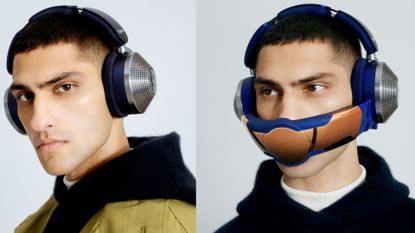The image comprises two juxtaposed square photos, each featuring the same young man in his early 20s with short hair, shaved on the sides. In the left photo, he stands against a light gray background, wearing a silver headset with black ear cushions and a black headband. His attire includes a tan coat with a black hood, and he has a serious expression while looking directly at the camera. In the right photo, set against a slightly darker gray background, he wears the same headset but with bright blue ear cushions. This headset includes a distinctive bronzed face mask attachment that covers his mouth and nose, resembling a Star Wars fighter pilot helmet. His clothing in this image consists of a white t-shirt under a black hoodie. His facial features include dark hair and eyebrows, and he has a lighter skin tone. The headset is highlighted as a Dyson air purifier filter model, characterized by its three-piece cushioned head strap and blue ear cups with a pronounced silver ring.